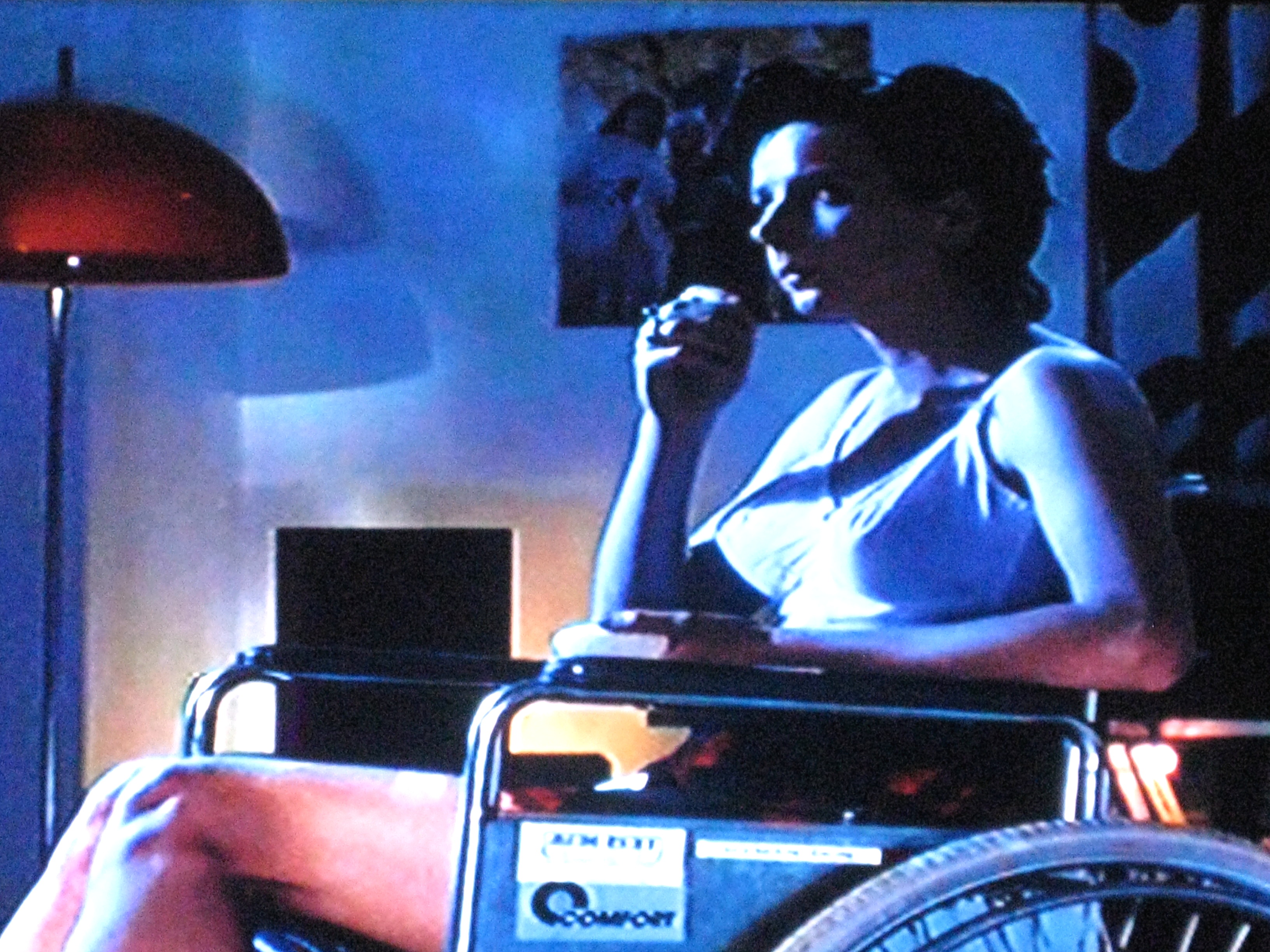The image appears to be a cinematic still, featuring a woman with short brown hair sitting in a wheelchair inside a dimly lit room with a blue hue, suggesting it could be a nighttime scene. She is dressed in a sleeveless tank top and is seen with her right arm raised, possibly snacking or smoking a cigarette, while her left arm rests on the wheelchair's arm. The wheelchair has a distinct square frame, with a sticker that seems to read "comfort" on its side. To her left, there is a prominent standing lamp with a red dome-shaped lampshade casting a warm glow. In the background, a retro-style picture hangs on the wall, and a speaker is placed near the lamp. The room is enveloped in shadows, adding to the scene’s moody and possibly eerie ambiance. The colors in the scene include pink, white, maroon, light blue, gray, silver, and black. Her legs extend towards the left, and she seems to look off to her left with a somewhat serious expression.